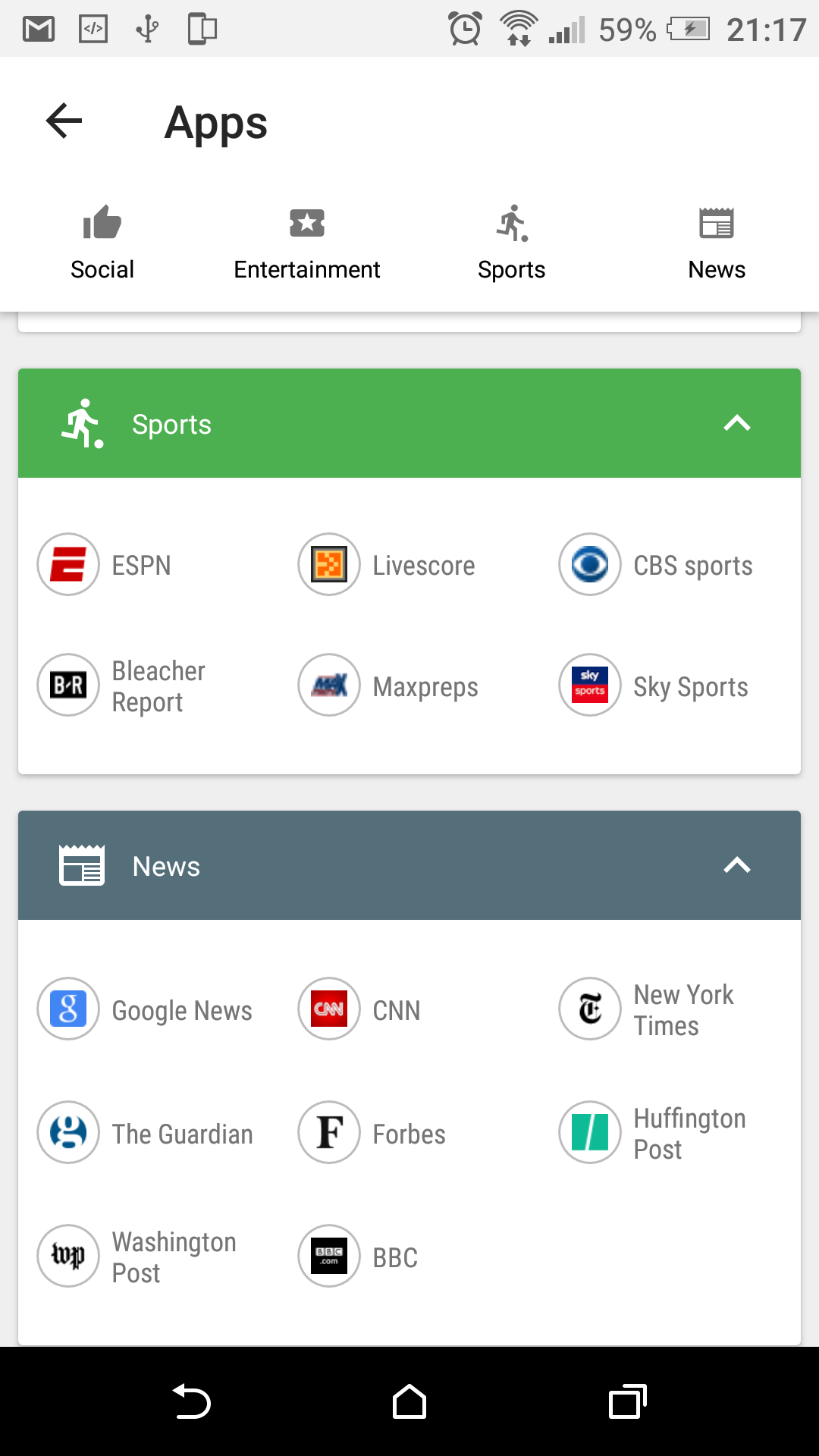This image is a screenshot of a smartphone displaying a section dedicated to organizing apps. At the top, there's a header titled "Apps." Below the header, there are four categories showcased by distinct icons: Social, Entertainment, Sports, and News, arranged from left to right. 

Directly beneath these category icons, there's a green bar with white text that reads "Sports." This section features six circular icons, each displaying the logo of a sports-related app, along with corresponding names next to them.

Following the Sports section, there's a gray bar with white text that says "News." This part showcases eight apps, similarly represented by circular icons with their logos at the center and their names listed alongside.

At the very bottom of the screen, a black bar features three icons, likely for navigation or additional functions. The structured layout and clear categorization make it easy to navigate through various app groups.